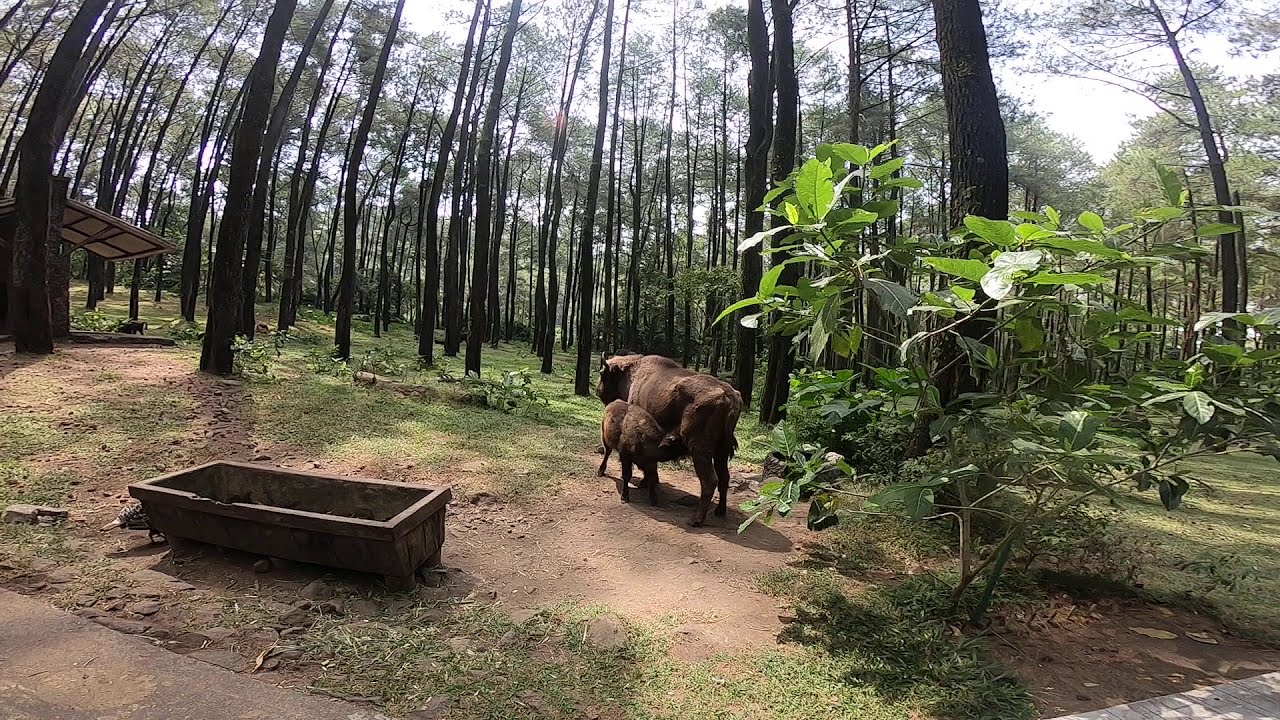In this daytime photograph, set within a serene forest, a picturesque scene unfolds. Towering trees with ample space between their trunks stretch towards the blue sky, which is peppered with clouds. The ground is a mix of lush green grass and brown soil, dotted with various plants and small shrubs with vibrant green leaves. Central to the image are two brown cows—a nurturing mother and her calf. The calf is seen drinking its mother's milk, suggesting a tender moment of maternal care. To the left, a cuboidal concrete container, possibly for water or dirt, stands nearby. Additionally, a hut-like structure with an overhanging roof sits in the background, adding to the rustic charm. The scene likely captures a spontaneous, authentic moment in nature, highlighting the peaceful coexistence of wildlife and the forest's verdant beauty.